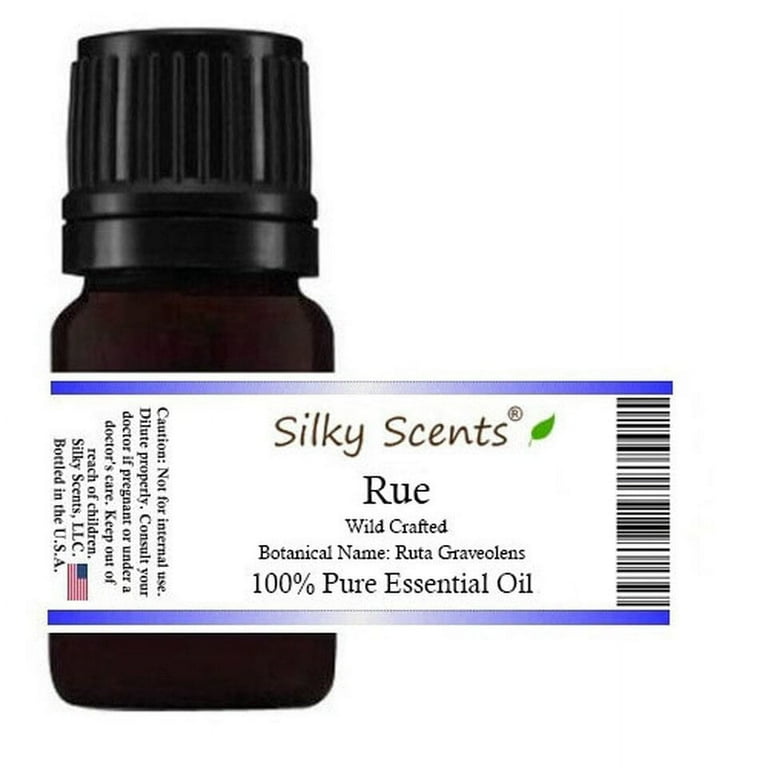This product image features a small, brown, square glass bottle typically used for essential oils, with a black ridged twist-off cap. The bottle is likely displayed on an online retail platform like Amazon, given the low-fi quality of the photo. The primary focus of the image is the label, which stretches from left to right and appears to be partially unattached on the right side, suggesting this might be an illustration rather than an actual photograph.

The label is white with blue lines running across the top and bottom, and prominently displays the brand name "Silky Scents," accompanied by a green leaf logo. The essential oil inside the bottle is RUE, which is indicated as wildcrafted. The botanical name listed is Ruta Graviolens, and the product is marked as 100% pure essential oil. The right side of the label features a barcode running vertically, while the left side includes a cautionary statement: "Not for internal use. Dilute properly. Consult your doctor if pregnant or under a doctor's care. Keep out of reach of children." The label also notes that the product is bottled in the USA, with a small American flag next to this information.